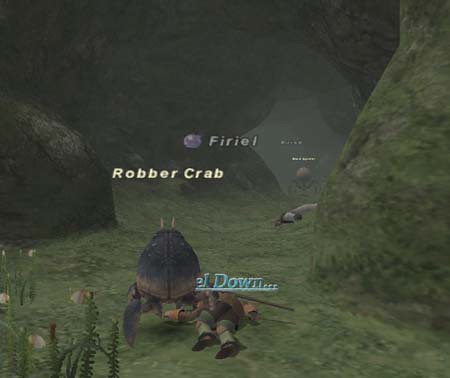In this nostalgic screenshot from Final Fantasy XI, a character is seen lying prone on the grassy ground of a pixelated, vibrant green area. In the foreground, a menacing Robber Crab stands over the player character, whose status is ominously indicated by the text "down..." The scene is set within a tunnel, where clusters of plants adorn the ground, adding to the fantasy atmosphere. Deeper into the tunnel, another Robber Crab is visible, along with a distinct purple blob symbol labeled "F.I.R.I.E.L." In the far background, additional text can be faintly seen, though it remains illegible. The overall setting evokes a sense of adventure and danger, characteristic of the game's immersive environments.